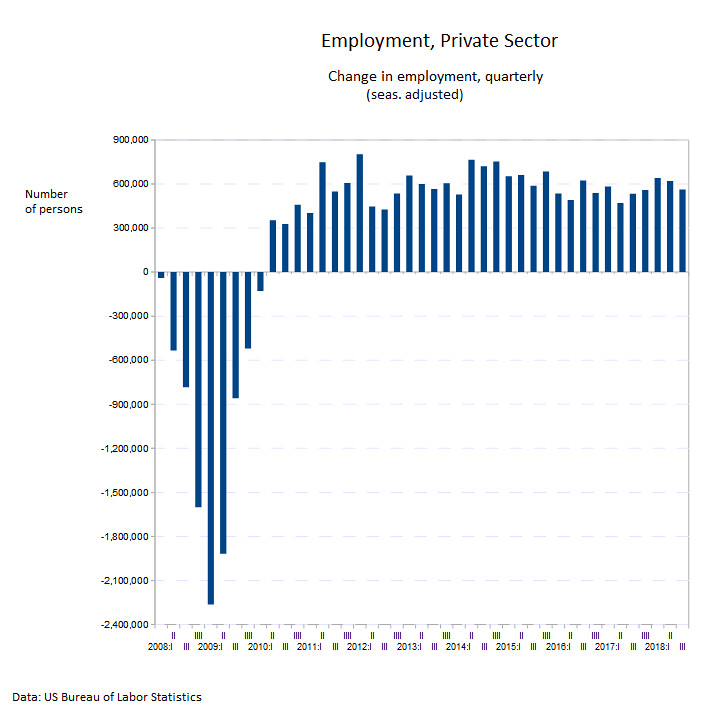The image is a detailed bar graph that illustrates the quarterly change in employment within the private sector, with data sourced from the U.S. Bureau of Labor Statistics. Titled "Employment Private Sector" at the top in black font, the graph further specifies "Change in Employment Quarterly (Seasonally Adjusted)." The bars representing the employment changes are blue against a white background, with the labels on the x-axis denoting years from 2008 to 2018, and the y-axis indicating the number of persons ranging from -2,400,000 to 900,000. Significant fluctuations can be observed: prior to 2010, most bars dip below zero, with the lowest point reaching nearly -2,400,000, whereas post-2010 bars generally ascend above zero, peaking close to 800,000. This graph vividly captures the employment trends, showing a stark contrast between the periods before and after 2010.